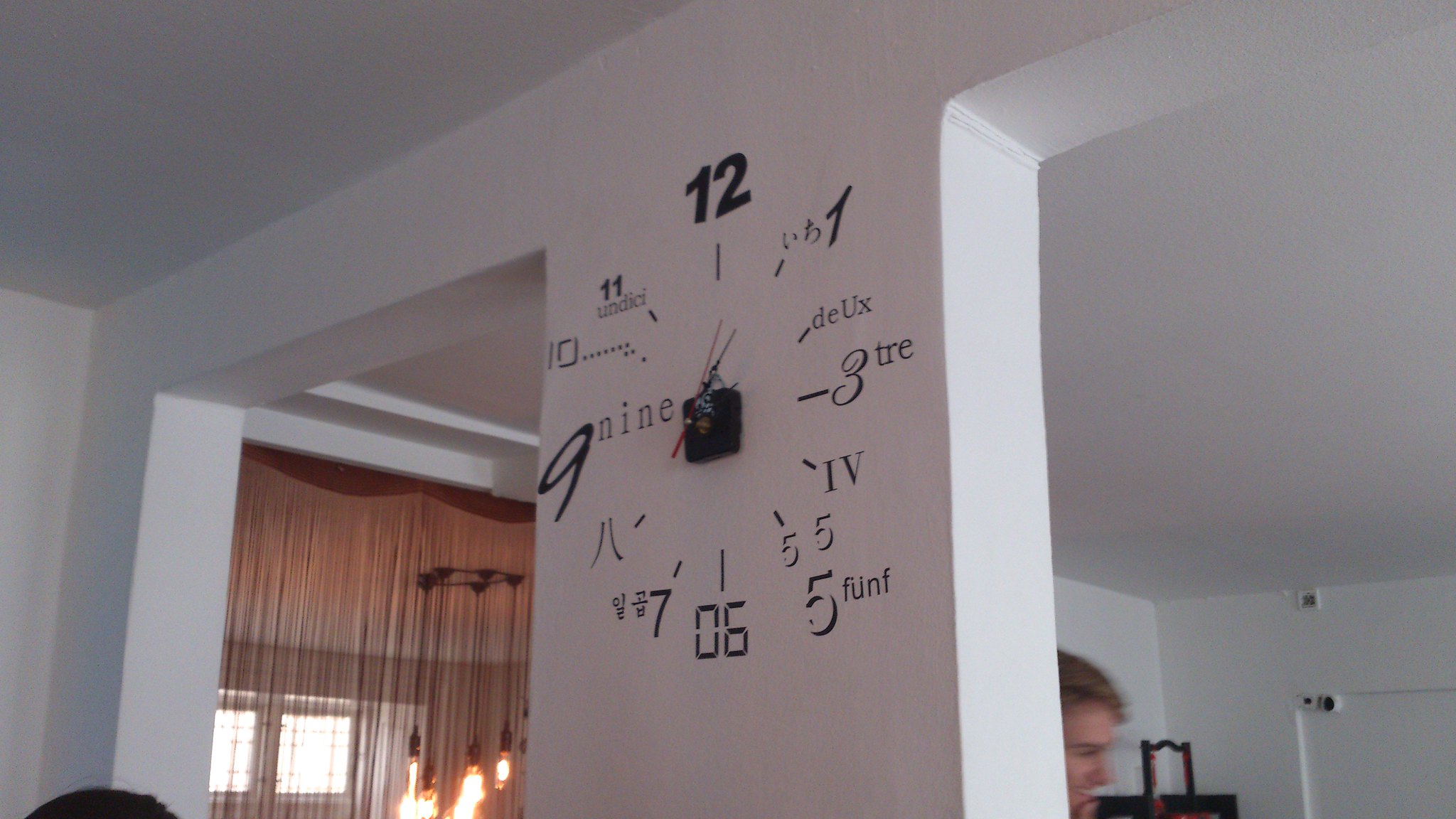This image captures a unique artistic installation within a white-walled room, featuring a clock painted directly onto a structural frame between two doorless pathways. The frame itself is also white, harmonizing with the minimalist interior. Each numeral on the clock is presented in a creatively unconventional manner:

- The number 12 is bold.
- The number 1 is styled differently.
- The number 2 is represented by the word "deix" in a foreign language.
- The number 3 appears as "3" with the adjacent text "tre".
- The number 4 is depicted using the Roman numeral "IV".
- The number 5 is written thrice alongside the word "FUNF".
- The number 6 is depicted in a digital format, as "06".
- The number 7 features Chinese characters next to it.
- The number 8 is shown with two symbols from another language.
- The number 9 is paired with the text "9".
- The number 10 follows in the same style as 9.
- The number 11 is written normally with some word beneath it.

In the background, visible through the pathways, two separate spaces can be seen. On the left, there are curtains bathed in light, and a chandelier with low-hanging lights adds a touch of elegance. On the right, a young, blonde-haired man with fair skin peeks into the frame, adding a human element to the scene. The entire setting is characterized by its stark white walls, enhancing the distinctiveness of the painted clock.